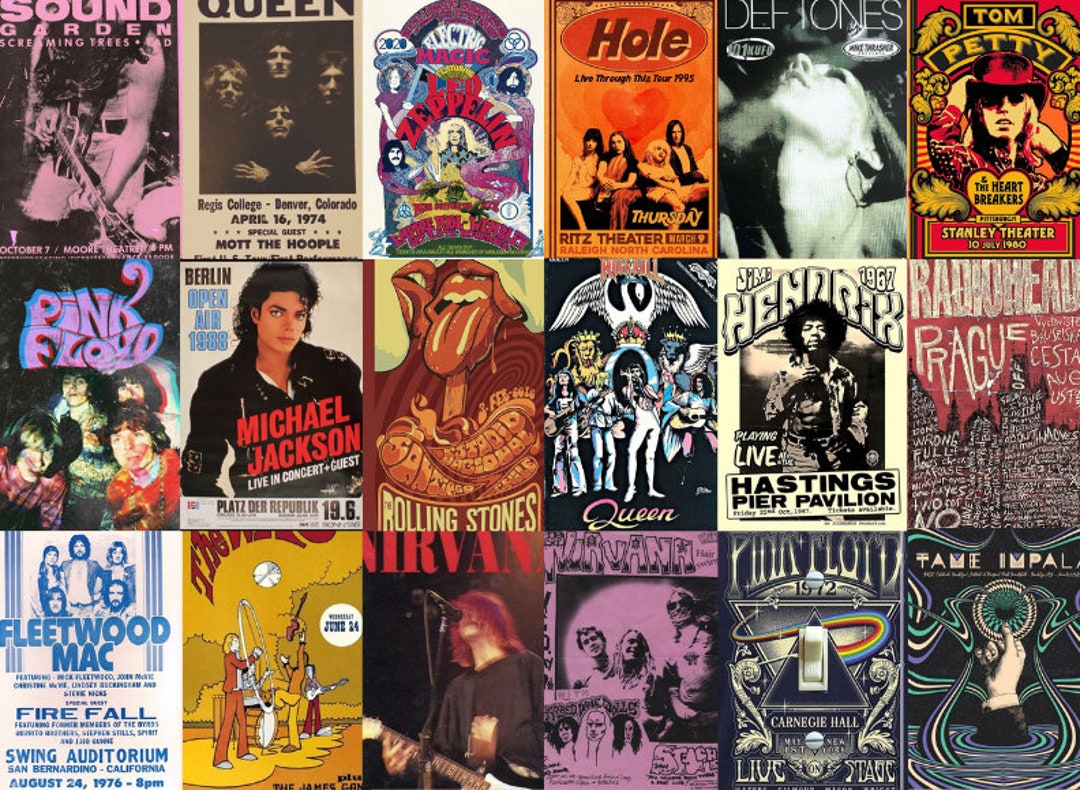This image showcases a vibrant collection of 18 colorful concert posters organized in three rows of six. Each poster vividly captures the essence and iconic imagery of legendary bands and artists. The top row features a pink Soundgarden poster, a Queen poster from 1974, a Led Zeppelin poster, a striking orange Hole poster, one for the Deftones, and Tom Petty and the Heartbreakers at the Stanley Theatre dated July 10, 1980. The middle row includes posters for Pink Floyd, Michael Jackson, the Rolling Stones, another Queen poster, Jimi Hendrix, and Radiohead with a Prague mention. The bottom row displays a blue and white Fleetwood Mac poster for an event at Firefall Swing Auditorium on August 24, 1976, a yellow poster of The Who, two Nirvana posters (one of which is pink), another Pink Floyd poster, and Tame Impala. Each poster not only announces the concert details but is adorned with images or motifs emblematic of each artist.